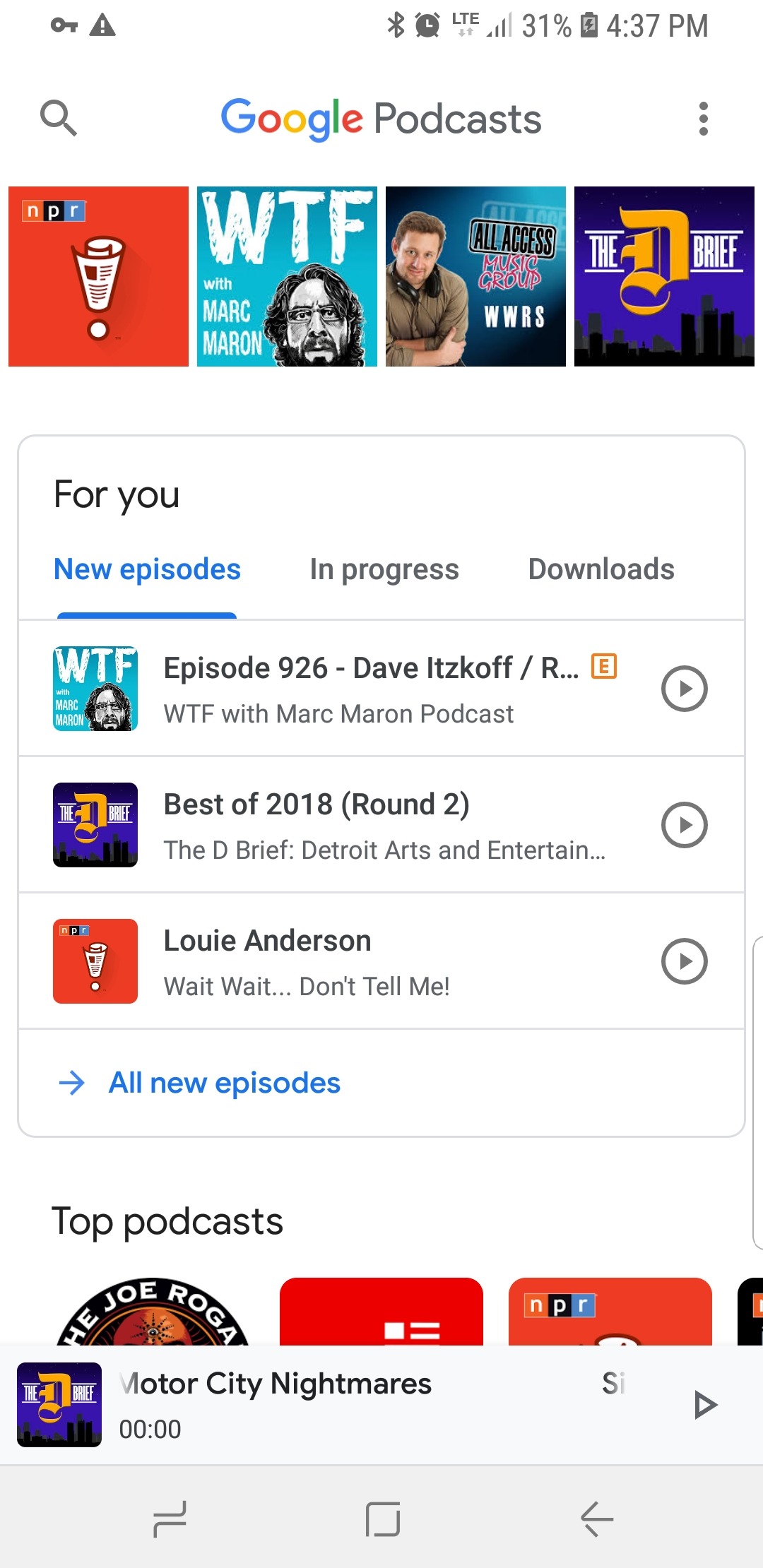This is a detailed screenshot of a Google Podcasts playlist. At the top, the Google Podcasts header is prominently displayed. Below it, four square thumbnails are arranged in a row, each representing a different podcast. 

The first thumbnail is NPR, featuring an exclamation point crafted from a rolled-up newspaper with a white dot. The second thumbnail is for Marc Maron's podcast, "WTF". The third thumbnail represents "All Access," and the fourth and final one on the right is for "The Debrief".

Underneath these thumbnails, there's a menu bar with options: "For You," "New Episodes," "In Progress," and "Downloads," listed from left to right.

The playlist showcases three episodes:
1. "Episode 926" from the Marc Maron podcast featuring David Itzkoff.
2. "Best of 2018, Round Two" from The Debrief.
3. "Louie Anderson" from "Wait, Wait, Don't Tell Me."

An arrow pointing to the right next to the text "All New Episodes" is highlighted in blue, suggesting more episodes can be accessed. At the bottom, more top podcasts are visible, although they are partially cut off.